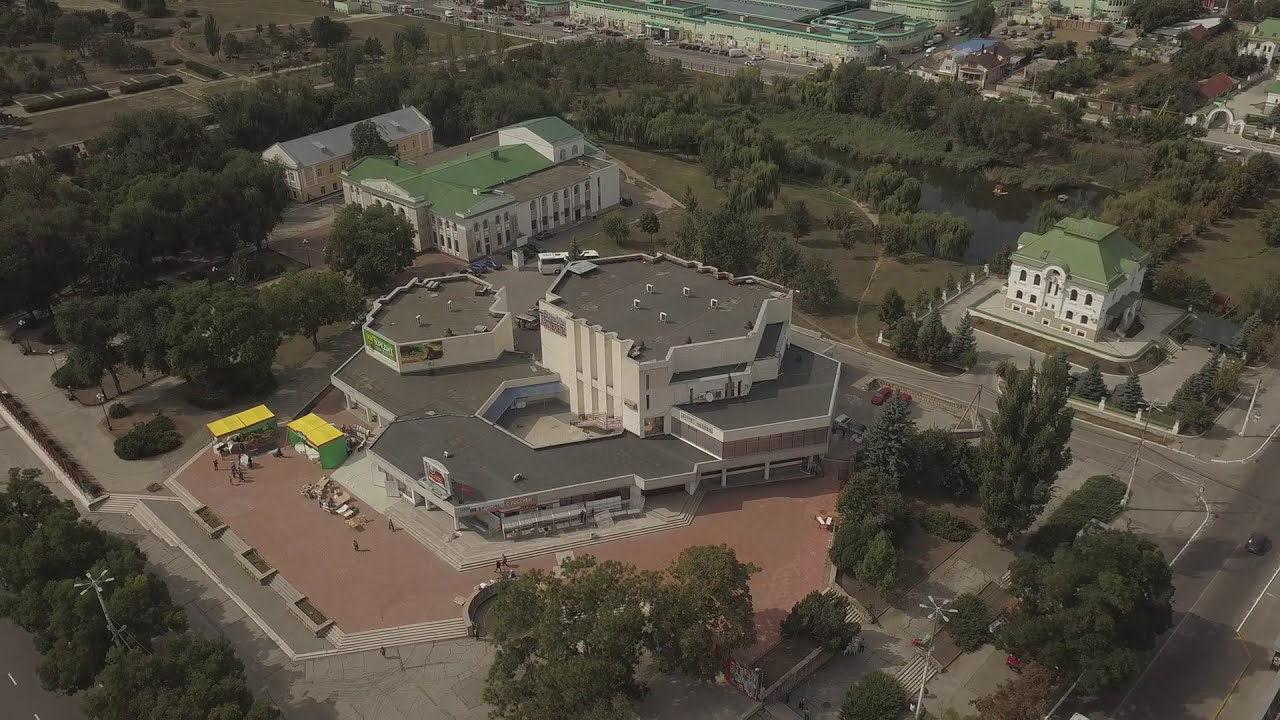This image presents an aerial view of a complex campus setting, potentially a city landscape or a university. The central focus is a large, round, multi-level building surrounded by a concrete walkway where people are seen walking. The walkway features yellow awnings or tents. This primary structure is part of a larger array of buildings, some with green roofs and others with flat black roofs, forming various polygonal shapes. Notably, the ground is covered with paved bricks. The campus is interspersed with several established trees and a pond area situated to the back right. Smaller buildings are visible throughout, with something resembling two yellow rectangles—possibly little tables for conversation—located in the lower-left corner. Roads encircle the buildings, tying the entire layout together.